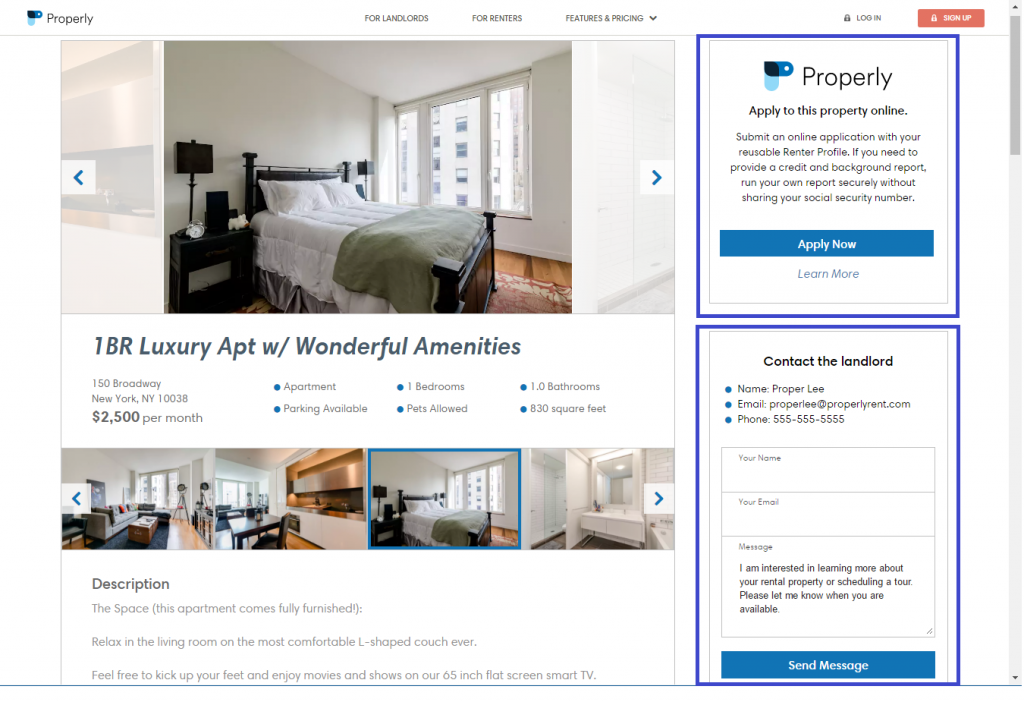Here's a detailed and cleaned-up caption for the image of the web page:

---

Screenshot of a real estate listing for a luxury apartment located at 150 Broadway, New York, NY 10038. The web page features a centrally placed image of a tastefully decorated bedroom. Key details of the apartment are prominently highlighted:
- **Rent**: $2,500 per month
- **Size**: 830 square feet
- **Rooms**: 1 bedroom, 1 bathroom
- **Amenities**: 
  - Fully furnished, including a living room with a plush L-shaped couch
  - 65-inch flat-screen smart TV
  - Parking available
  - Pet-friendly

The listing encourages prospective tenants to apply online using a reusable renter profile. It also specifies that applicants should run their own credit and background checks securely, without sharing their social security number. Contact information for the landlord is provided, including an email (properly@properlyrent.com) and a phone number (555-555-5555). A form for inquiries is also available, where interested parties can express their interest and request further information or schedule a tour.

The web page has a clean, white background with black text for easy readability.